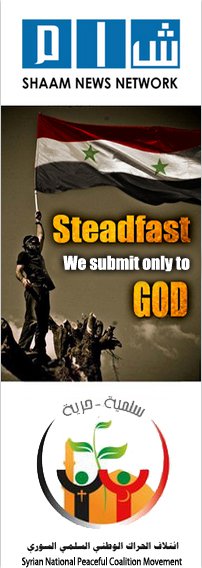This is an image of an advertisement from the Shaman News Network. The advertisement, in a long rectangular format, features several detailed elements. At the top, there is a blue logo composed of three blue squares, each containing letters: D, I, and W, followed by the text "Sham News Network." Below this, there is a photograph of a soldier standing on a mountain or rock, who is holding up a red, white, and black Syrian flag with three green stars on the white stripe. The flag bears the inscription "Steadfast, we submit only to God." The soldier is dressed in black, with a black t-shirt, black pants, and a black mask covering his face.

Beneath the photo is a white square featuring a round circle divided into black and red sections, with two cartoon figures standing at the bottom. The black figure, which has a cross on its chest and a round circle for a head, holds its arms up. Next to it, the red figure has a crescent moon on its chest and a green circle for a head, also with arms raised. They are jointly holding a large green stem with three green leaves. Behind these figures is an image suggestive of a mosque. Below this scene, there is script that appears to be in a Middle Eastern language, and under this script, the text reads "Syrian National Peaceful Coalition Movement."

This advertisement appears to be a pamphlet promoting a peace movement in Syria and is presented by the Shaman News Network, emphasizing a coalition for national peace.